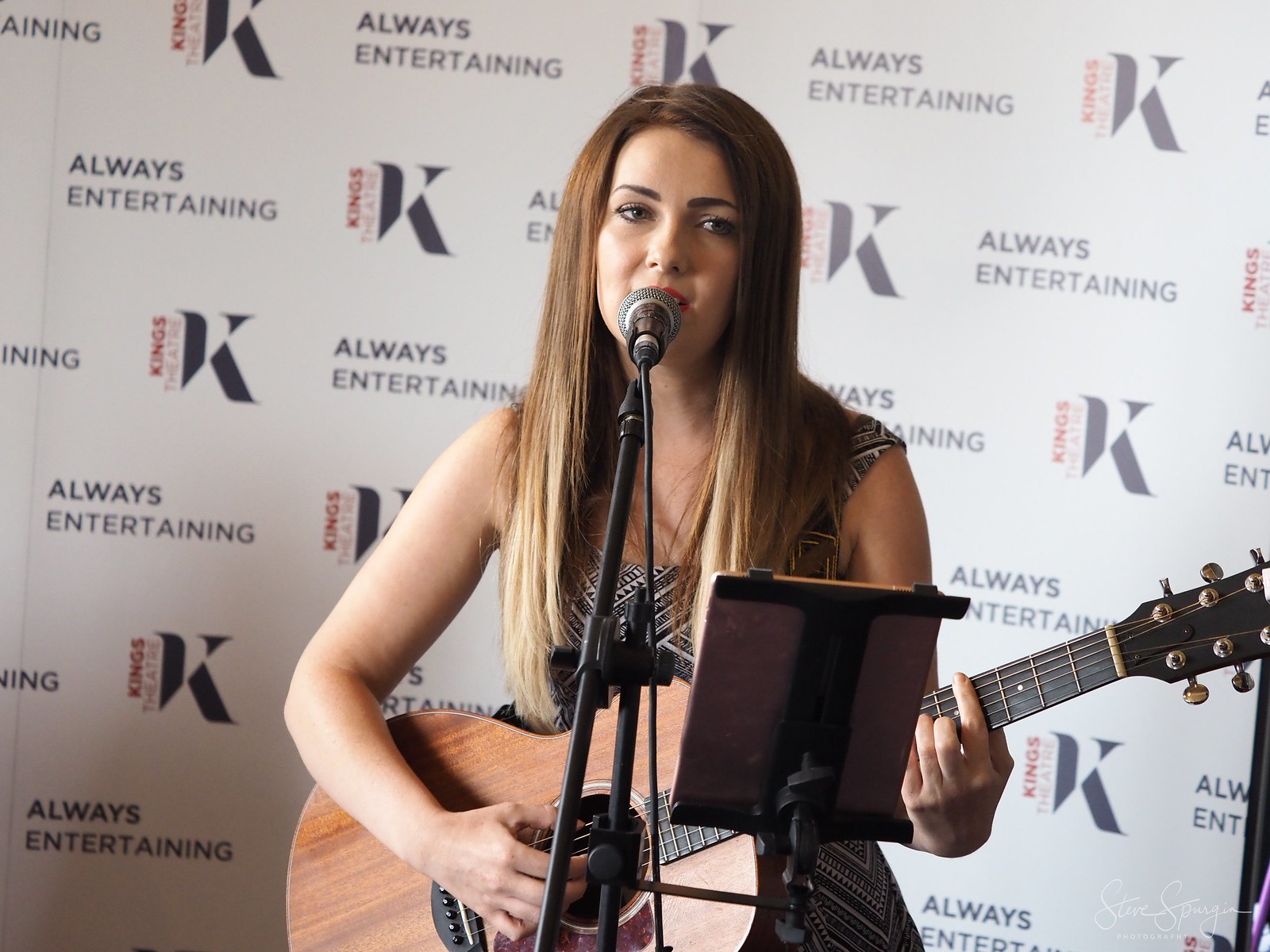In the center of this image, a young Caucasian woman with long, straight brown hair featuring blonde tips, dressed in a sleeveless black and white geometric print dress, is seated and playing an acoustic wooden guitar. With her left arm supporting the guitar's dark brown or black neck and her right hand strumming the strings, she appears to be performing. A microphone on a stand is positioned directly in front of her, close to her red-lipsticked mouth, suggesting she is singing. She gazes slightly off to her left, giving the impression of being deeply immersed in her music. In front of her is a small music stand which could possibly hold music sheets or a tablet, though she is not looking directly at it. The backdrop is a white banner with a repeating pattern that reads “Always Entertaining” and features a large letter "K" followed by the words "Kings Theater." This finely detailed setting captures the essence of a live, intimate musical performance.